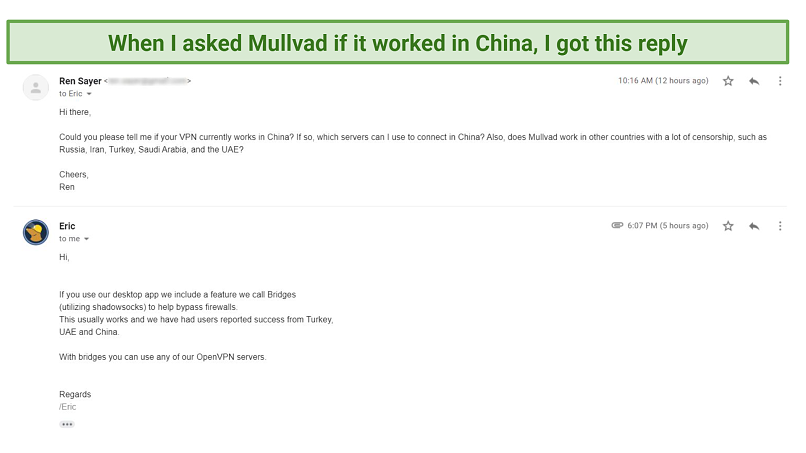In the image, there is a conversation depicted between two individuals discussing VPN functionality in countries with heavy internet censorship. At the top, there is a query from a user named Ren Seiya addressed to Eric asking if their VPN service, MOVA, operates in China and other heavily censored countries like Russia, Iran, Turkey, Saudi Arabia, and the UAE. Ren wants to know which servers can be used to connect from China. In response, Eric describes a feature in their desktop app called Bridges, which uses Shadowsocks to bypass firewalls. Eric notes that this feature has been successful for users in China, Turkey, and the UAE, and it allows access to any of their OpenVPN servers. The exchange highlights the VPN's potential efficacy in censorship-heavy regions.